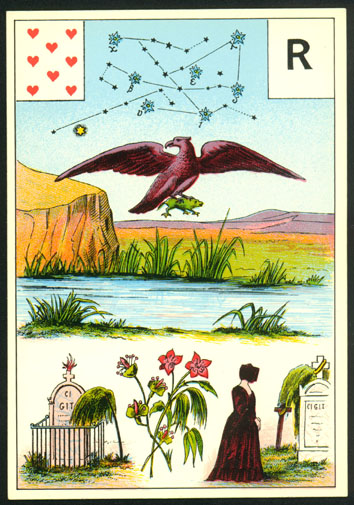The image is a vertically oriented illustration framed with a thin black border, followed by a slightly thicker off-white border, and finished with another thin black line, which encapsulates the detailed scene within.

In the upper left-hand corner is a playing card adorned with eight red hearts, but without any numbers. Opposite to this, in the upper right-hand corner, a single, large capital letter 'R' is prominently displayed in black. Between these two corners, a blue sky dotted with a series of interconnected points creates a kind of daytime constellation.

Beneath this upper section, the main focus of the image reveals a massive brown bird with its wings spread wide horizontally, positioned as if flying towards the left (nine o’clock direction). The bird clutches a green rodent in its talons. To the left of the bird, a rugged brown cliff is visible with patches of grass below it, extending downwards to meet a stretch of plains which then transition into a backdrop of distant mountains.

As the viewer's eye moves downward, a river flows horizontally from left to right, set against the lush green land adorned with grass and foliage. 

In the lower portion of the image, specifically on the left-hand side, a fenced-in gravestone is surrounded by pink flowers. To the right of this gravesite stands a lady in a long purple dress, gazing at another gravestone, adding a poignant human element to the serene yet complex landscape.